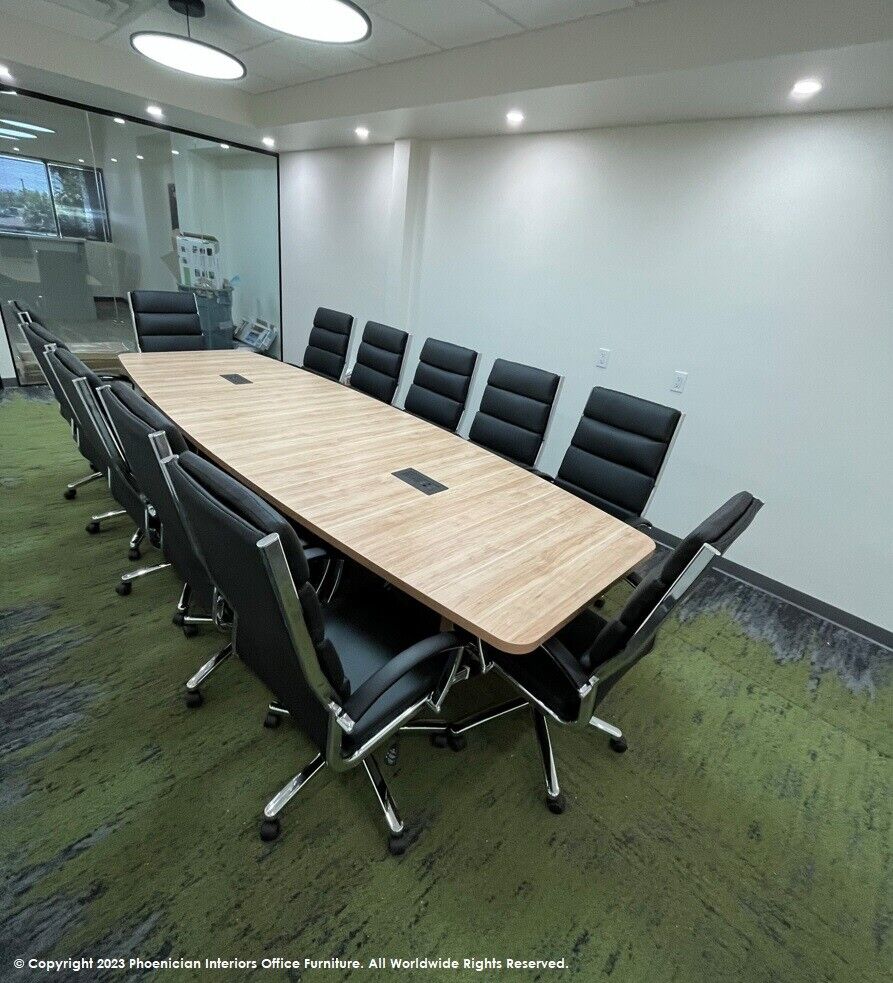The image depicts an indoor conference room with a notably tranquil and professional atmosphere. Central to the room is a long, rectangular wooden table, surrounded by a total of twelve black leather chairs—five on each side and one at each end. The floor features a distinctive green carpet, evoking a moss-like texture. The room's walls are white, and it is illuminated by large fluorescent lights on the ceiling. Clear glass doors at the back of the room offer a view into adjacent areas, suggesting an open and interconnected office environment. Notably, the image is marked with a copyright notice from "Phoenician Interiors Office Furniture, 2023," indicating that this setup is part of their product line.